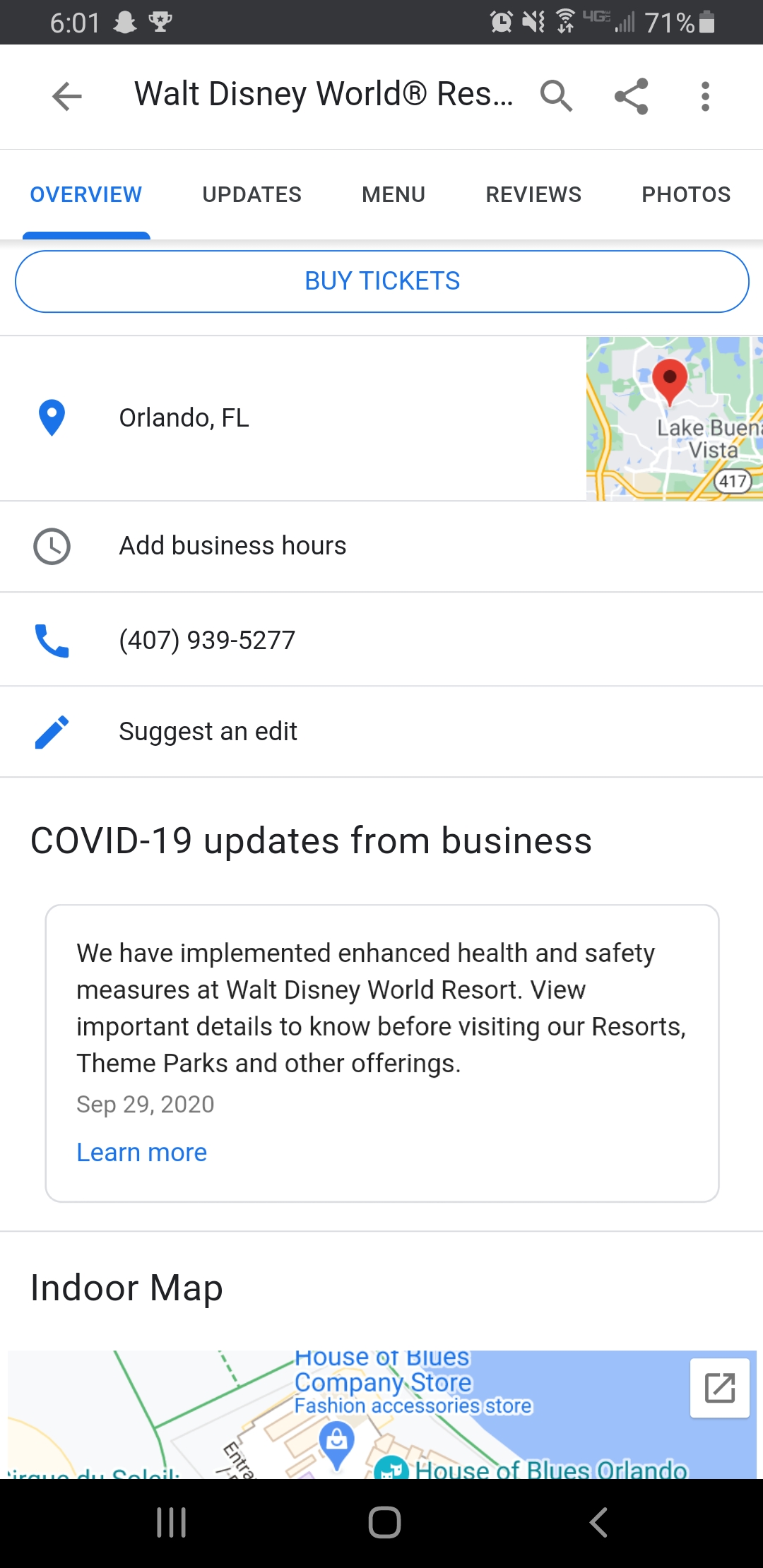**Detailed Description of a Walt Disney World Reservations Tablet Screenshot:**

The image displays a tablet screenshot of the Walt Disney World Reservations interface, structured for purchasing tickets. Against a clean, white background, the black block header prominently reads "Walt Disney World RES...". At the top of the interface are several navigation tabs: "Overview" (highlighted in blue as the selected option), "Updates", "Menu", "Reviews", and "Photos".

Beneath these tabs, a wide "Buy Tickets" button stretches across the full width of the page, presented in blue block print. Below this button, there are four lines of bold text followed by various informational elements. 

The first line includes a location pointer icon indicating "Orlando, Florida" to the left, accompanied by a thumbnail map on the right. The second line invites users to "Add business hours". The third line features a phone icon followed by the contact number "407-939-5277". The last line in this section contains an option to "Suggest an edit", implying the information on the page may not be complete.

There is also a highlighted COVID-19 update from the business, stating: "We have implemented enhanced health and safety measures at Walt Disney World Resort. A few important details to know before visiting our resorts, theme parks, and other offerings." This update is dated September 29th, 2020, with a "Learn More" link in blue text below it.

At the bottom, an indoor map is partially visible, seemingly truncated to only show the top of the "House of Blues Company Store" but missing the lower part of the map.

Overall, the screenshot provides a navigation-friendly layout for users to access and manage their reservations and other relevant information for Walt Disney World.